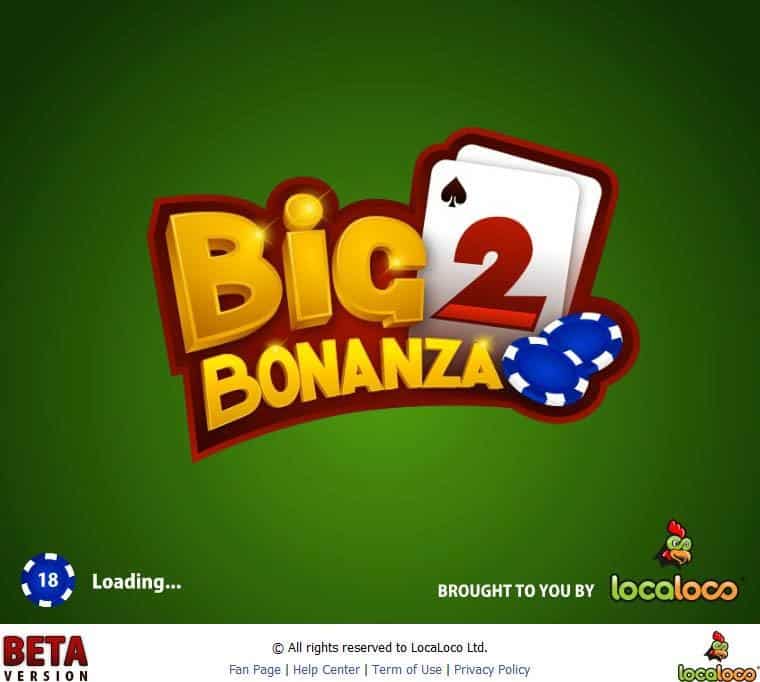The image is an advertisement for an online game, featuring a vivid green square background with slightly darker shading in the upper corners. Dominating the center of this square is the bold, three-dimensional gold text "BIG" in large block letters with a dark red border, and beneath it, in smaller gold uppercase letters outlined in red, is "BONANZA". To the right of "BIG" is a stack of two playing cards, with the top card displaying a large red number 2 and a black spade symbol on a white background. Below and right of the cards, two poker chips in blue and white are positioned. 

In the lower left corner, there is another blue poker chip marked with a white "18". Adjacent to this chip, the word "LOADING..." is written in white. On the bottom right, the text "BROUGHT TO YOU BY" appears in white, followed by the company name "LOCA LOCO" in green and orange, adorned with a smiling rooster logo above it. 

At the bottom of the image, within a white section, "BETA VERSION" is displayed prominently with "Beta" in red over a smaller black "version". Below this, small black text lists legal and help sections including "COPYRIGHT ALL RIGHTS RESERVED TO LOCA LOCO LIMITED," "FAN PAGE," "HELP CENTER," "TERMS OF USE," and "PRIVACY POLICY." Another "LOCA LOCO" logo with the rooster is featured in the bottom right, solidifying the brand's presence.